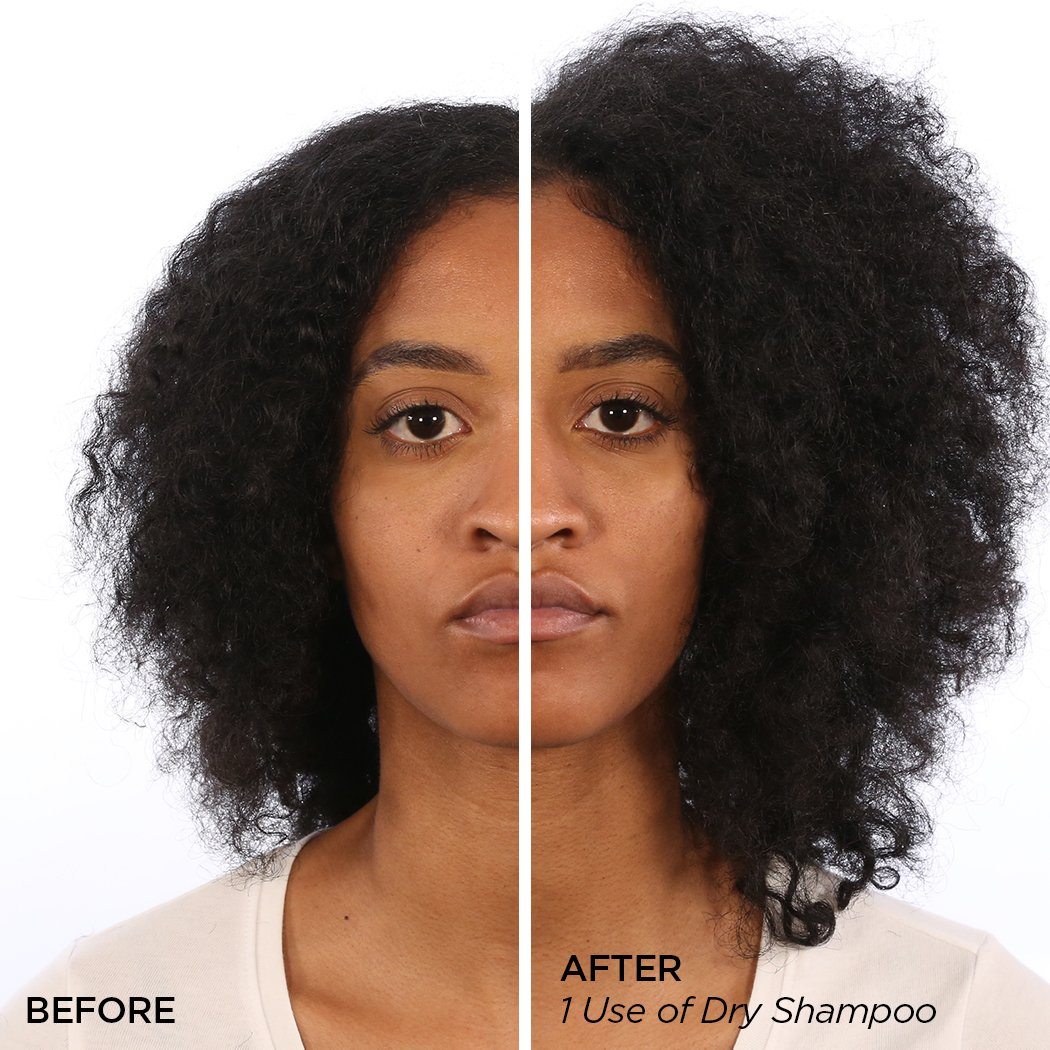The image is a before-and-after advertisement photograph featuring an African-American woman, likely in her 20s or 30s, with medium brown skin and black, curly hair. The photograph is divided into two halves by a white line with a white background. On the left side is the "before" image, where her curly hair appears flatter and more relaxed. On the right side is the "after" image, showcasing the effects of one use of dry shampoo, with her hair looking significantly more voluminous, fluffy, and vibrant. The woman has a serious expression, staring directly at the camera. She is wearing a light-colored top, identified as either beige or pale lilac by different observers. The text accompanying the image is in black font. This side-by-side comparison effectively highlights the transformative impact of the dry shampoo on her naturally curly hair.